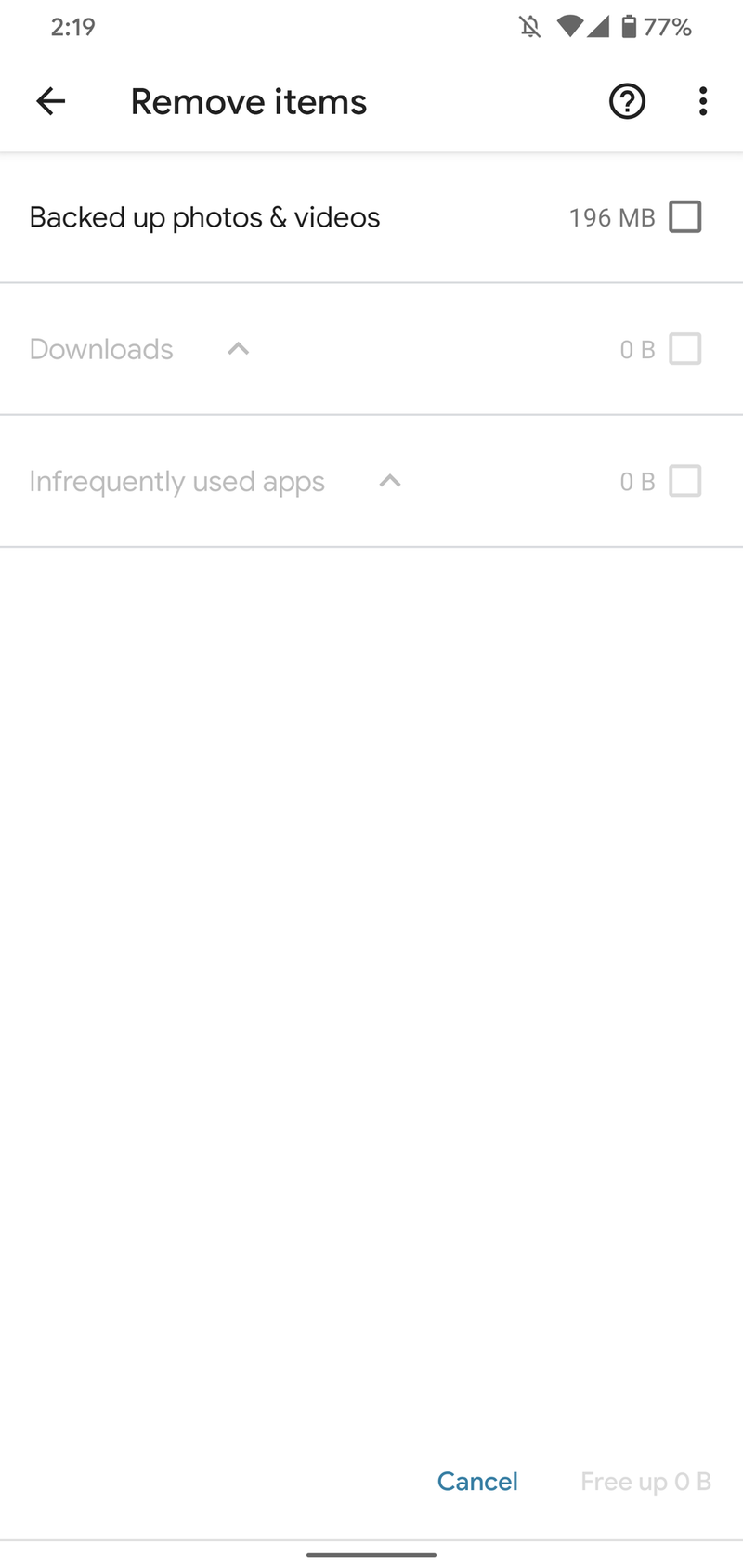**Detailed Caption:**

The image depicts a screen with various system notifications and interface elements. 

1. **Top Left Corner:**
   - A small page icon with the number "219".

2. **Top Right Corner:**
   - A notification bell icon followed by the word "Druid".
   - A cone icon and a 90-degree triangle.
   - A battery icon showing a 77% charge level.

3. **Second Row, Left to Right:**
   - An arrow pointing left.
   - The phrase "Remove items".
   - A gray circle with a question mark inside.
   - Three vertical dots.

4. **Below the Second Row:**
   - A horizontal line spanning from left to right.

5. **Section 1:**
   - Text: "Backed up photos and videos, 196 MB".
   - An unchecked checkbox.

6. **Section 2:**
   - A horizontal line.
   - Text in very light gray: "Downloads, 0B" with an up arrow next to it.
   - An unchecked checkbox.

7. **Section 3:**
   - A horizontal line.
   - Text: "Infrequently used apps, 0B" with an up arrow next to it.
   - An unchecked checkbox.

8. **Bottom Section:**
   - A horizontal line spanning the width of the screen.
   - In the middle of this line, a smaller dark gray line.
   - Above this, the text "Cancel" in blue and "Free up to 0B" in light gray.

The page seems to be part of a storage management or cleanup interface, indicating space usage and options for freeing up space.